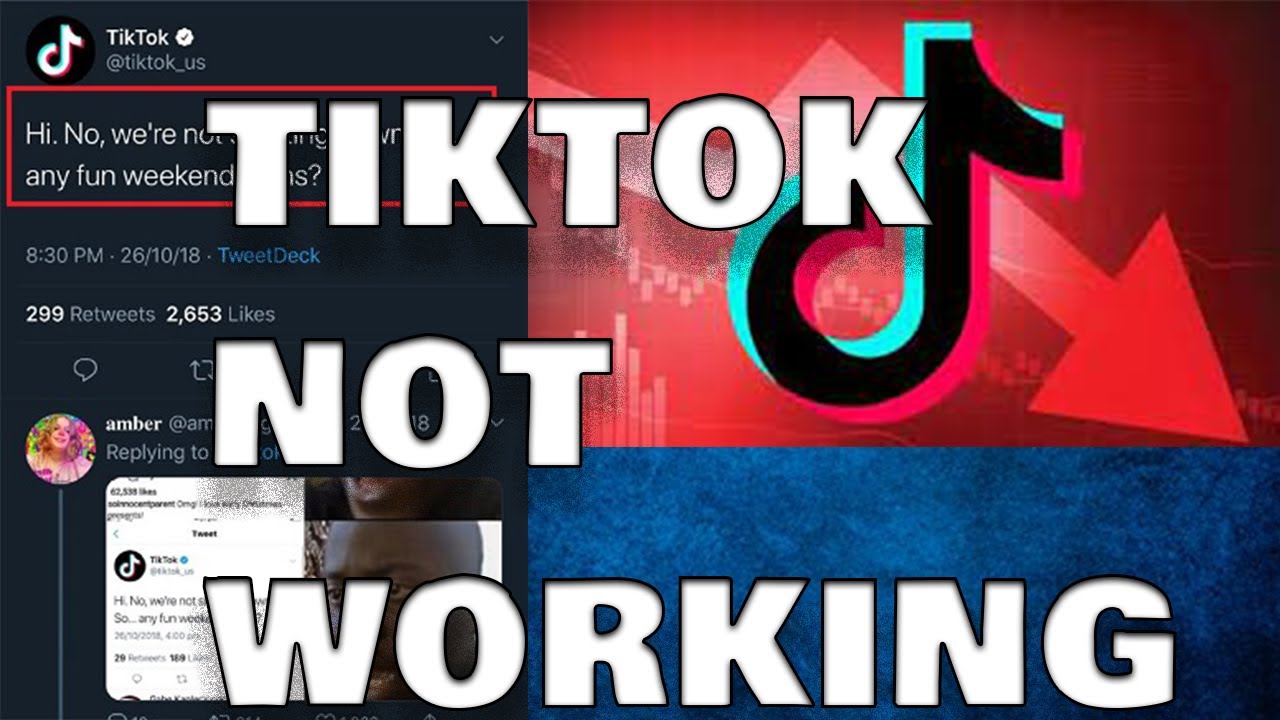The image is a screenshot from a website with a predominantly black background on the left side. At the top of this section, there is the TikTok logo consisting of a stylized musical note and the text "TikTok" next to it. Below the logo, it reads "@TikTok_US" accompanied by a circular icon with a black checkmark inside, indicating a verified account. 

To the right of this, there is a dropdown arrow. Further down, some partially obscured text reads "We're not..." which is highlighted by a red outline. 

The timestamp on the post is marked as 8:30 PM, October 26, 2018, followed by "TweetDeck" written in blue font. Beneath this, the engagement metrics show 299 retweets and 2653 likes.

Additionally, there is a circular profile icon with an image of a person named Amber next to some partially visible text. An overlay that says "TikTok not working" obscures this section.

On the right side of the image, the background transitions into a red top half and a blue bottom half, separated diagonally by a red arrow pointing down from the red section to the blue section. At the top right, there is a black TikTok logo contrasting against the red background.